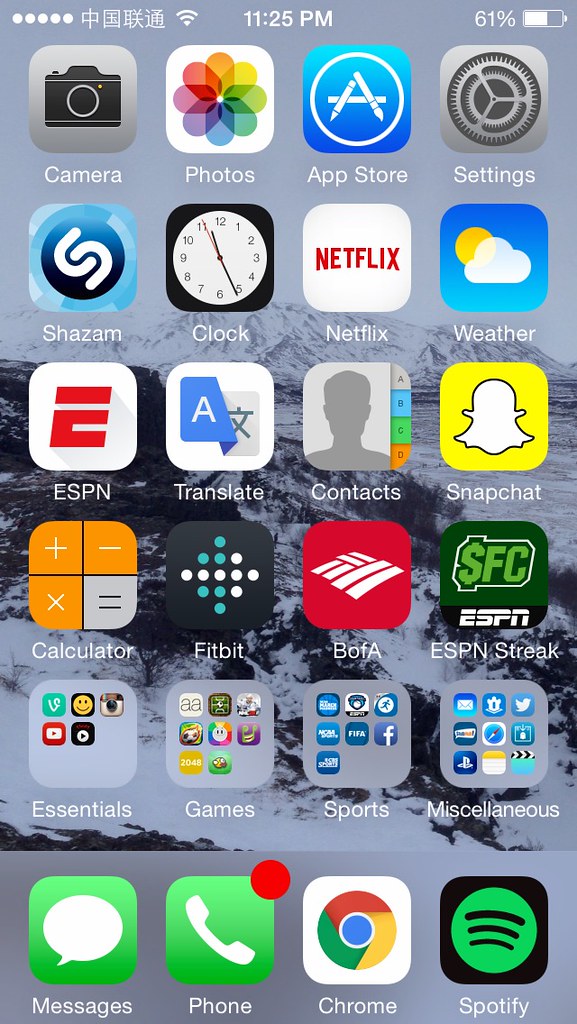In this screenshot of a smartphone's home screen, the display showcases various app icons organized neatly into rows. At the very top, the status bar indicates the time as 11:25 p.m., and the battery level at 61%, indicated by the battery icon. The first row of apps includes Camera, Photos, App Store, and Settings. Moving to the second row, we see Shazam, Clock, Netflix, and Weather. The third row houses ESPN, a translation app, Contacts, and Snapchat, identifiable by its distinctive yellow and white icon. The fourth row features Calculator, Fitbit, Bank of America (labeled as BOA), and the app Streak. Below these rows, there are folders labeled Essentials, Games, Sports, and Miscellaneous, each containing additional apps. The bottom-most row includes essential apps for daily use: Messages, Phone, Chrome browser, and Spotify. The background image is a serene winterscape, depicting mountains in a grayish hue, exuding a calm and peaceful ambiance.